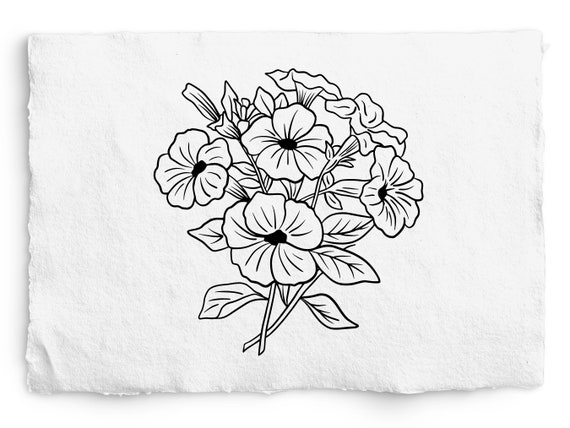The image depicts a piece of white, slightly fibrous, Arts and Crafts-style paper with frayed, rough edges, suggesting it might be either a torn-out or folded paper towel or napkin. This paper sits on a white background, giving it a monochromatic, clean appearance. Central to the paper is a detailed, black-and-white line drawing of a bundle of flowers, resembling a bouquet. The flowers are intricately designed with four to five fully opened petals per flower, accompanied by partially visible budding flowers in the background. The stems and leaves are also visible, contributing to the bouquet-like arrangement of the flowers, which include bell-shaped bodies that add depth and texture to the drawing. The entire image lacks any text, focusing solely on the natural beauty of the floral illustration.